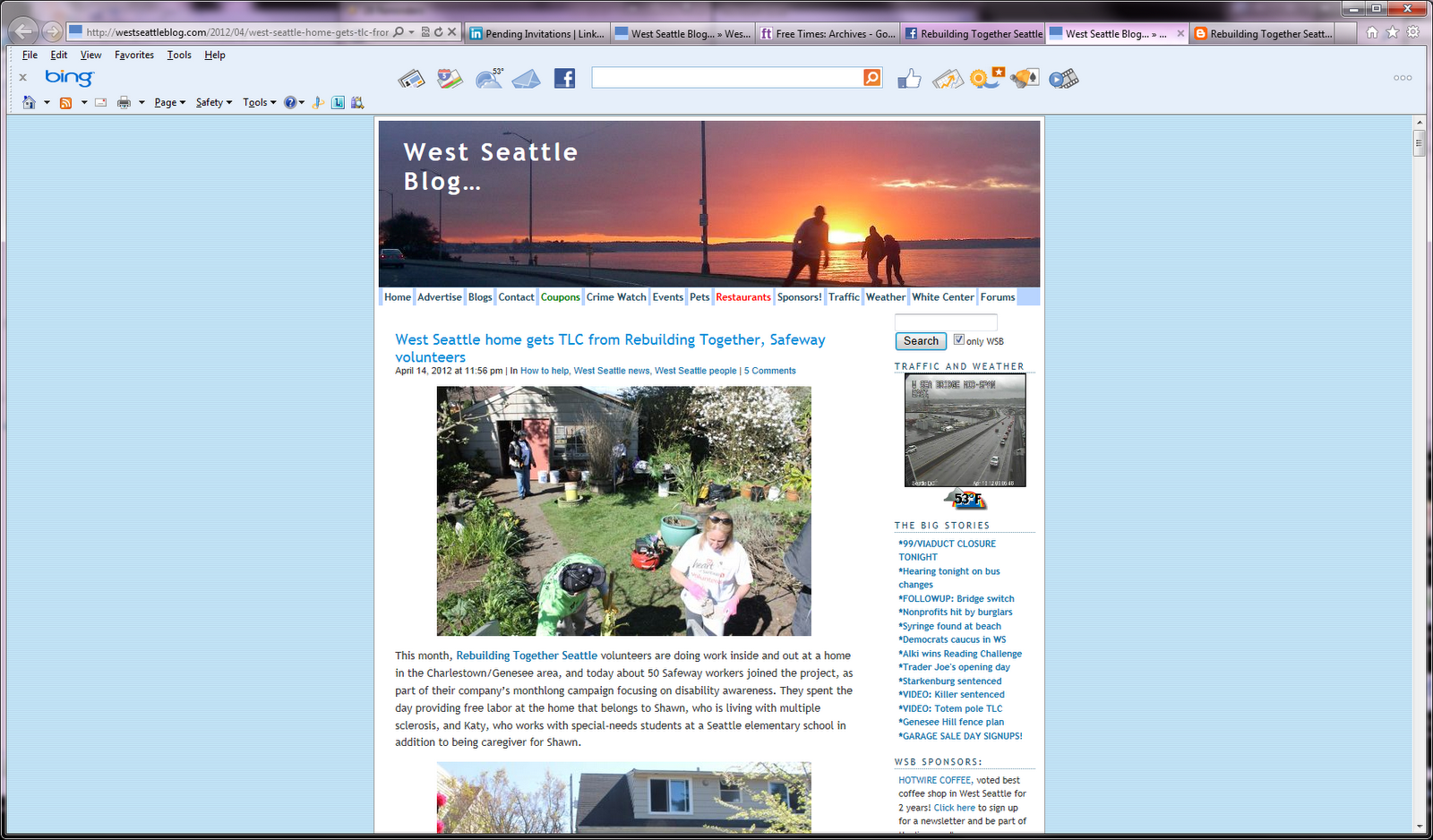A detailed and organized screenshot of a West Seattle blog displayed on a computer screen through Bing. The background of the interface is a light baby blue. At the top of the screen, there are several navigation elements placed from left to right: a back arrow, a forward arrow, a search bar, and seven tabs.

The main content area of the blog begins with a prominent rectangular banner showcasing a stunning sunset over water. The banner features an intense and vibrant sky with hues of orange, red, and purple. In the center-right of the banner, three individuals can be seen gazing at the radiant sunset. Light poles extend from the center toward the left side of the image, contributing to the depth and perspective.

Beneath the banner is a navigation menu that includes quick links to various sections: Home, Advertise, Blogs, Contact, Coupons, Cruise Watch, Events, Pets, Restaurants, Sponsors, Traffic, Weather, White Center, and Forums.

The main page currently displays an article titled "West Seattle Gets TLC from Rebuilding Together and Safeway Volunteers," accompanied by relevant images and paragraphs detailing the event and volunteer efforts.

This thorough and engaging blog layout invites readers to explore the diverse content and stay informed about West Seattle's community activities and updates.